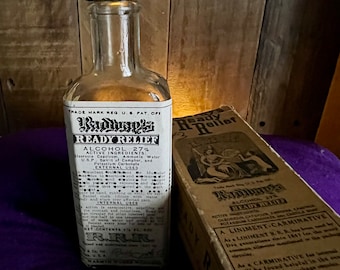This photograph features a historic medicinal artifact from the Western period of the United States. At the center is a glass bottle with a rectangular shape and a narrow top, missing its cap. The bottle has a white label with dark, stylistic lettering that reads "Radway's Ready Relief" and indicates it contains 27% alcohol. Promising to relieve various ailments, the label includes extensive, minuscule text. The bottle is set against a wooden wall. To its right is the worn, rectangular box it comes in, with light brown coloring. The box bears black letters stating "READY RELIEF" and features an antique black-and-white illustration of a woman and child. It’s labelled as liniment, indicating it’s used externally, likely applied to the skin. The photograph is completed with the setting on what seems to be a purple tablecloth under subtle lighting that accentuates the vintage liniment bottle and its packaging.